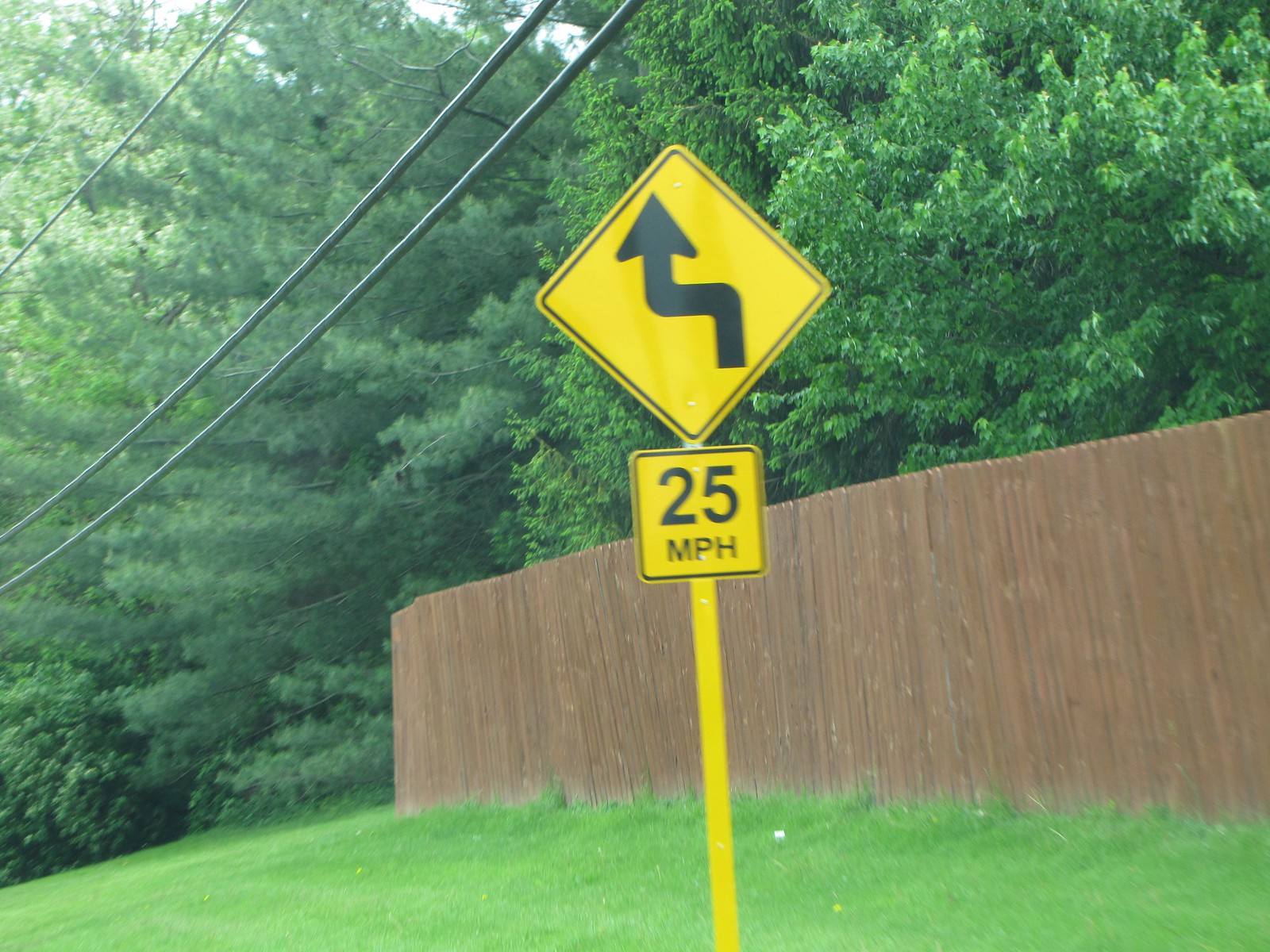A peculiar roadside sign is mounted on a yellow pole. The pole supports two signs: the lower one is a traditional square-shaped, yellow sign indicating a speed limit of 25 miles per hour. Above it, a much larger, diamond-shaped yellow sign features a convoluted black arrow. The arrow begins by pointing upward, then makes a sharp left turn, before pointing upward again and ending in a standard arrowhead. This suggests a complex change in direction ahead, resembling a route that first moves north, then turns left, and finally continues northwards, possibly indicating a twist or curve in the road. 

In the background, a wooden fence lines the edge of a neatly mowed grassy area. Overhead, cables run parallel to the fence, and beyond it, a dense forest of mature trees looms, adding depth and natural beauty to the setting.